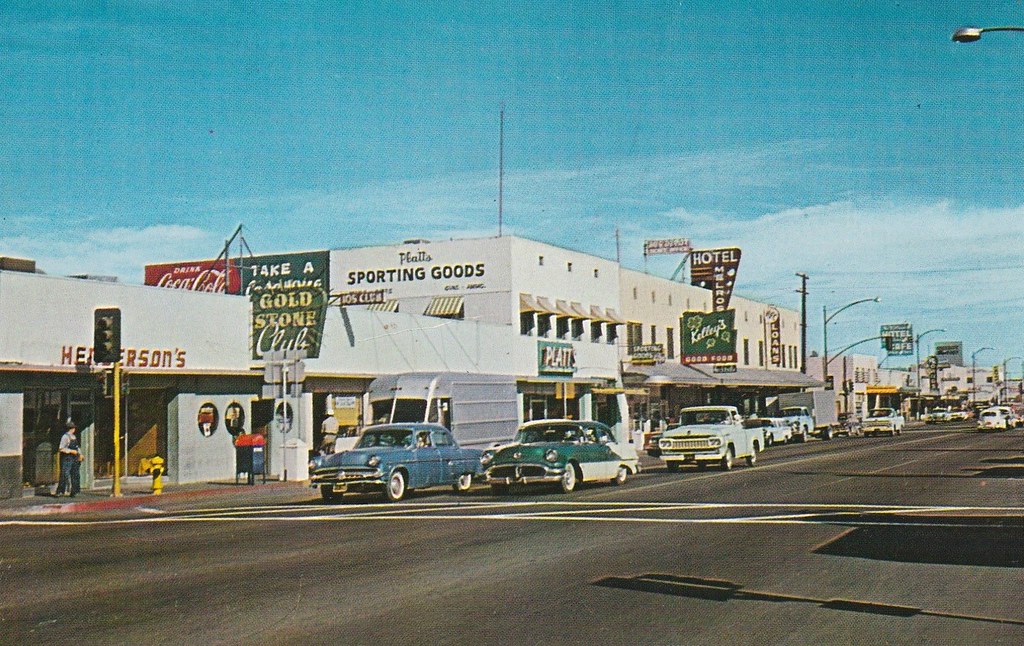The photograph appears to be from the 1950s or 1960s, captured in a downtown area with a vintage charm. The scene is dominated by classic cars with long fenders, rounded windshields, and white-rim tires. Notable vehicles include a blue car, a green and white car, and a baby blue pickup truck with a white cab. The street is an asphalt road with no visible potholes, lined with various shops and businesses that create a typical mid-20th-century street view. 

To the left, there’s a prominent white building marked "Henderson’s," where a woman is seen exiting, and a yellow fire hydrant stands in front. Further down are signs for “Platt’s Sporting Goods,” “The Goldstone Club,” and a red Coca-Cola advertisement partially visible with old-fashioned lettering. A hotel sign, possibly reading "Hotel Melrose," and a bar or food establishment called “Kelly’s” are also part of the streetscape. The storefronts are diverse, with some taller, some shorter, all forming a continuous block that gives a sense of a bustling main street.

The sky above is clear blue with some wispy, low-lying clouds. A streetlamp rises from the top right of the image, casting shadows down onto the scene, suggesting it’s a bright sunny day. A yellow streetlight pole and a mailbox also feature in the image, adding to the vintage urban feel. The overall picture not only highlights the architecture and vehicles of the era but also captures a slice of everyday life from a bygone period.